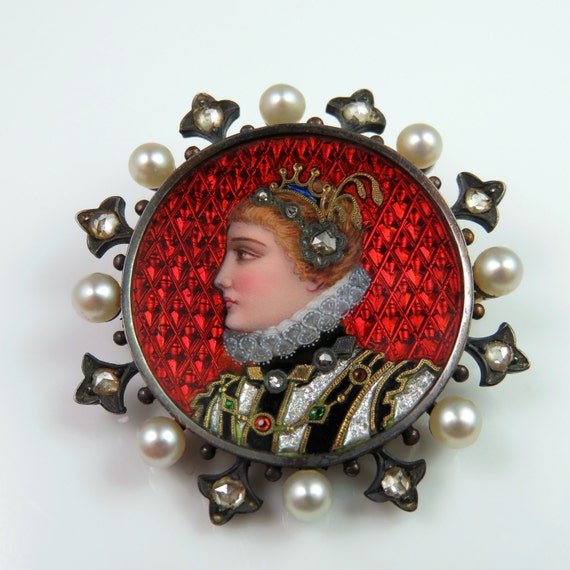The image displays a vintage brooch set against a solid white background. The brooch is round, framed by alternating pearls and metallic petal-like structures, some of which contain smaller pearls. The metal is a blackish-brown color. The central area of the brooch features a detailed portrait of a woman with red hair adorned with a crown and jewels in hues of green, red, blue, and ruby. The woman is dressed in an early 17th-century tunic with a high white collar, set against a background of two different wine shades—a light and a dark wine color forming a diamond pattern. The intricate detailing of the pearls and metallic elements adds an elegant touch to the overall antique aesthetic of the brooch.